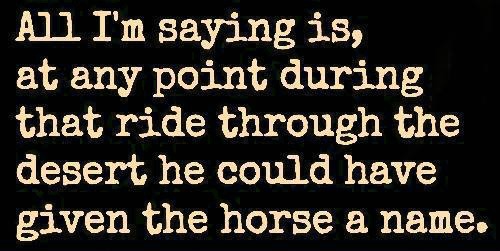This is a small, narrow rectangular digital image in landscape orientation, appearing to be a humorous social media post, possibly originating from platforms like Facebook, Instagram, or TikTok. The background is solid black, creating a stark contrast with the text, which is rendered in a decorative, typewriter-style font. The text is a creamy, off-white color, resembling an eggshell or light tan. The message reads: "All I'm saying is, at any point during that ride through the desert, he could have given the horse a name." This commentary humorously references the well-known song lyric, "I've been through the desert on a horse with no name," pointing out the ironic possibility of naming the horse during the journey.